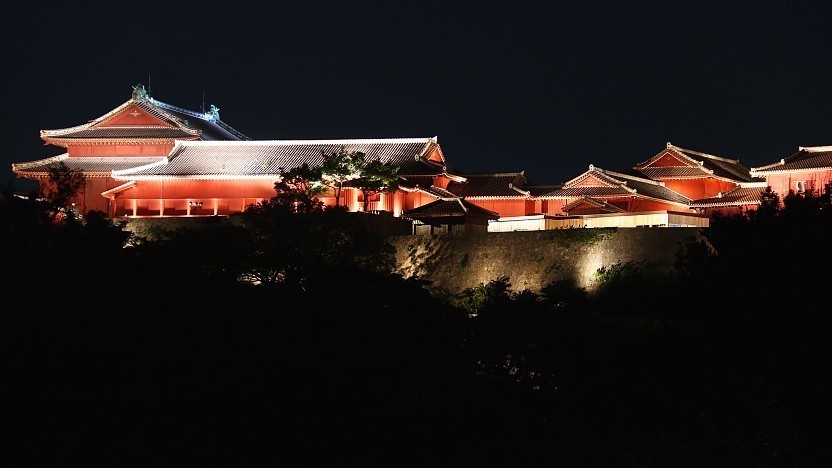This captivating night scene portrays a picturesque, walled compound nestled on a mountain, characterized by traditional Chinese architectural elements. The structure encompasses approximately eight interconnected red-brick buildings with peaked, A-framed roofs, noticeably illuminated by spotlights. The tallest central building is distinguished by its prominent white pillars. The entire compound is guarded by a tall stone wall, also brightly lit, and flanked by a dark forest in the foreground adding a mysterious ambiance.

Amidst the intricate layout, several details stand out: there appears to be a small white building in front of the compound and a structure resembling a guard tower behind the wall, suggesting an emphasis on security. One particularly intriguing feature is a man climbing a ladder on one of the roofs, illuminated by a spotlight. The scene is framed by a pitch-black sky, enhancing the dramatic and enchanting aura of this mountaintop retreat.